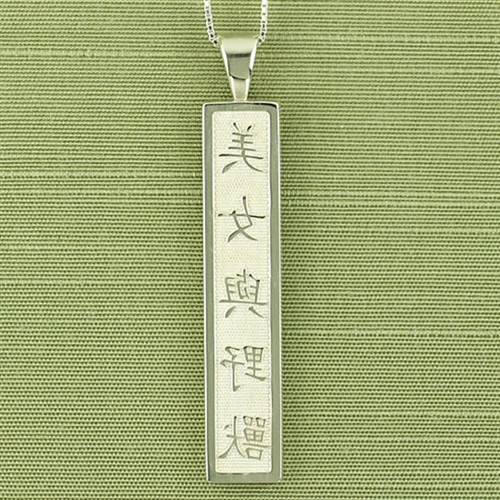The image depicts a horizontally rectangular necklace with a pendant, set against a textured light and dark green background that resembles a plastic tablecloth or woven fabric. The necklace features a fine silver chain with small loops, from which a long, oblong pendant hangs. The pendant has a creamy white background with a subtle greenish tint and is bordered by a silver frame. The front of the pendant displays five Chinese or Japanese block characters arranged vertically. There is a soldered silver piece at the top, through which the chain loops, allowing the pendant to hang. The textured background showcases threads running horizontally across, adding a layer of complexity to the image.